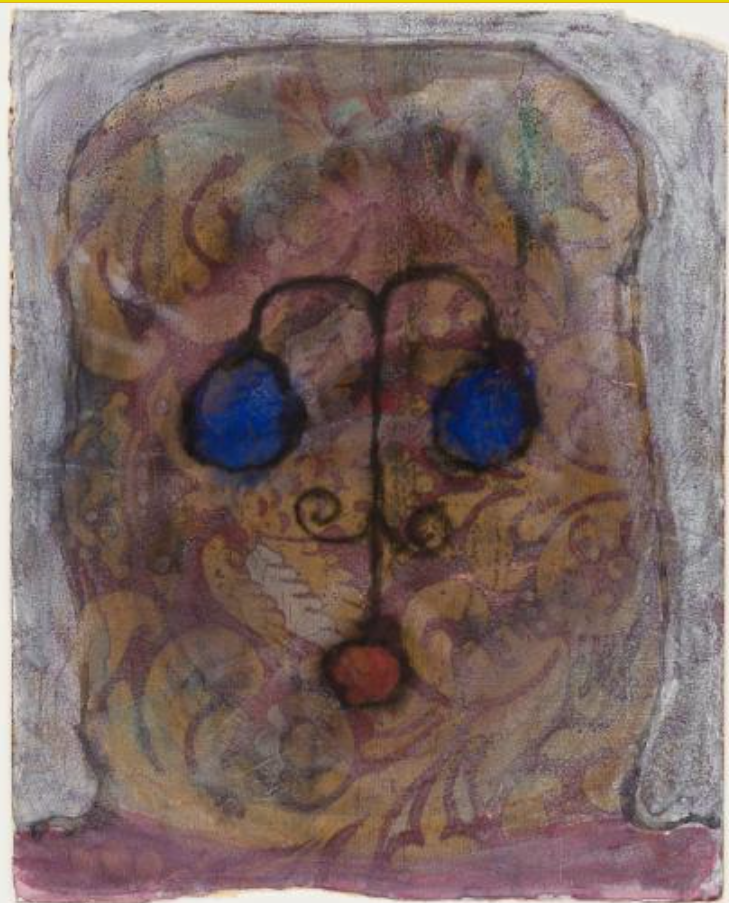The image is an abstract drawing or painting featuring a central object on a vaguely floral background with red and golden-yellow elements. The background transitions from reddish-pink with golden-yellow patterns resembling ornate scrolls or leaves to swirls of gray and white towards the edges. In the middle, a black bar with a skinny base curves outward to the right and left, ending in two blue circular shapes. Below this, at the bottom of the bar, there is a red circular shape. The design also incorporates a purple region at the bottom that blurs into the main area, contributing to the overall smudgy, abstract aesthetic. The central object and shapes create a composition that some might interpret as having a whimsical, almost street lamp-like appearance amidst the intricate backdrop.